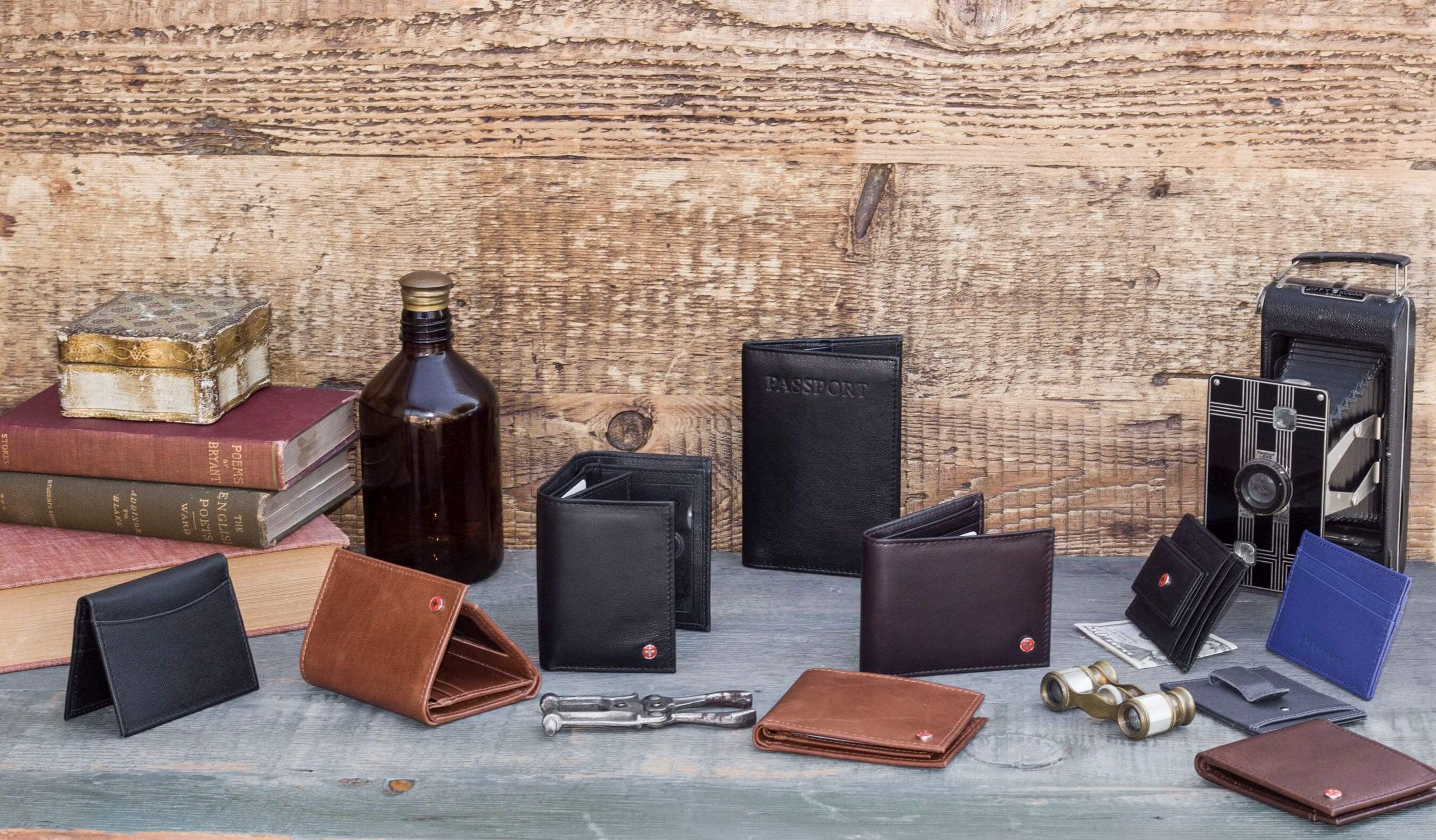The image showcases a clean and organized tabletop set in a rustic, old-world styled room, likely a home office or a store. Dominating the scene are various leather wallets in shades of black, brown, dark reddish-brown, and even silver, diligently arranged on a light gray, wooden table. The backdrop is composed of light brown, natural wood planks, enhancing the antique and masculine ambiance. To the left, there are three vintage stacked books in green, maroon, and gray, complemented by a dark growler-type jug with a gold cap. On the right, there's a classic black camera with a silver lens, possibly an accordion-style model, and a pair of antique binoculars. The overall setup is meticulous, evoking a sense of nostalgia and timeless sophistication.